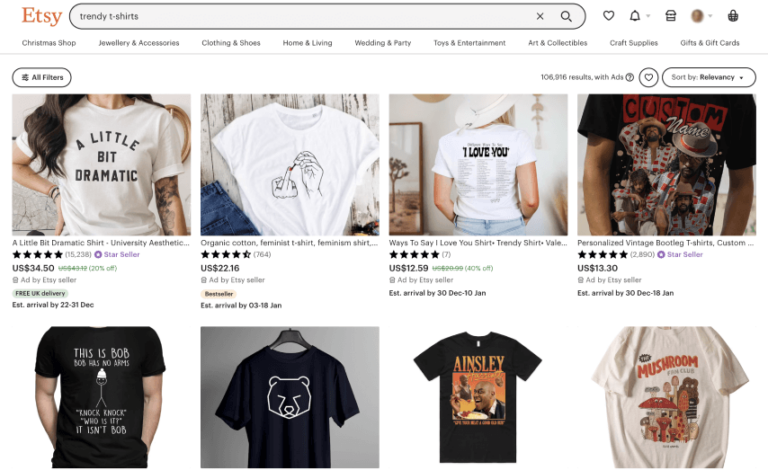This is a detailed screenshot of the Etsy website displaying a search for "trendy t-shirts." The Etsy logo, prominent in orange letters spelling out "E-T-S-Y," is located in the upper left corner. To the right of the logo, there's a search box where the phrase "trendy t-shirts" has been entered, leading to the current display of results.

The background of the page is a clean, flat white, highlighting eight different t-shirt listings in a grid formation. Each search result is presented in a distinct box, showcasing either an individual t-shirt or a model wearing it.

In the top row, the first t-shirt on the left is a white tee with the phrase "A Little Bit Dramatic" printed on it. Next to it, the second t-shirt features an image of a hand displaying the middle finger while applying red nail polish to the fingernail. The third t-shirt in the top row is adorned with the words "I Love You," followed by a block of smaller text that is unreadable in the screenshot. The fourth t-shirt, located on the far right of the top row, is a customizable black tee that allows users to add their own names and images.

Moving to the bottom row, the first t-shirt on the left is black and bears the simple phrase, "This is Bob." The second t-shirt from the left in the bottom row displays a bear face outline with the word "Ainsley," presumably referencing the Mem Ainsley meme. The final t-shirt on the right of the bottom row is black with the word "Mushroom" printed on it, accompanied by illustrations of mushrooms and other characters.

This screenshot effectively captures a diverse selection of trendy t-shirts available on Etsy, displayed in an easy-to-navigate format, with a mix of text, graphics, and customizable options.